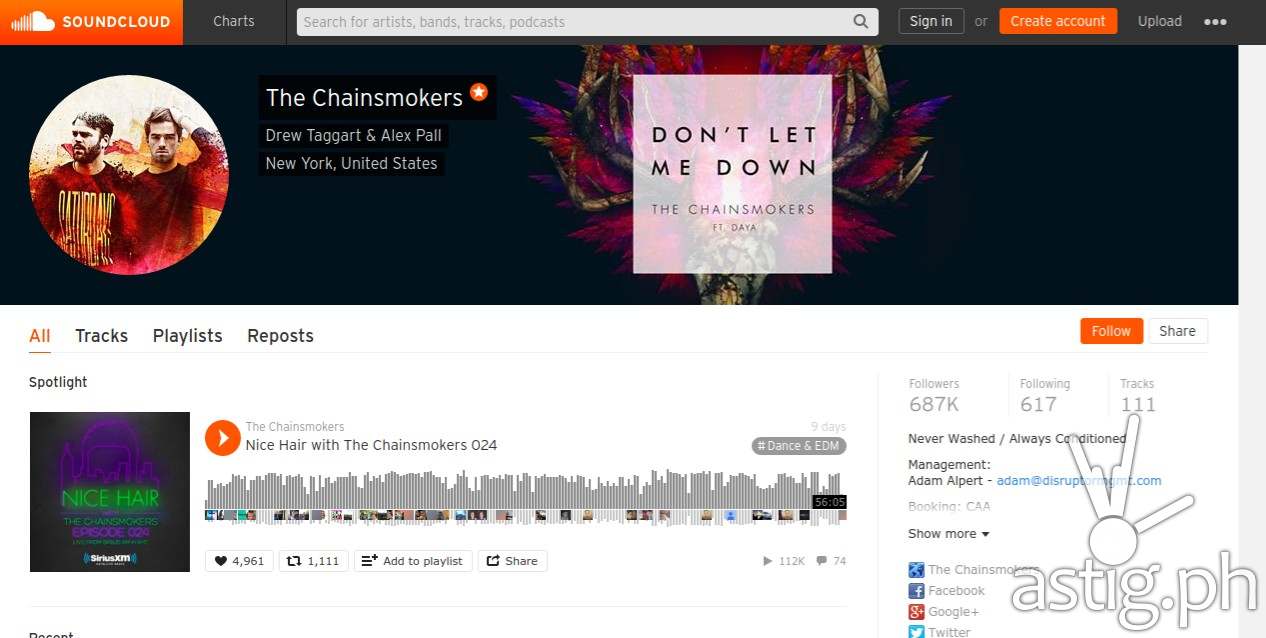This screenshot captures a segment of the SoundCloud website. At the top left, there is an orange rectangle with the SoundCloud logo, which consists of a white cloud icon followed by the word "SoundCloud" in white font. Positioned to the right of this, a gray rectangle features the word "Charts" in white font. Within this gray rectangle, there is a white search field containing the placeholder text "Search for artists, bands, tracks, podcasts" in gray font, along with a magnifying glass icon denoting its function.

Further to the right, options to "Sign In" or "Create an Account" are visible, followed by an "Upload" button.

Directly beneath this header section, there's a banner showcasing the musical duo The Chainsmokers. The banner confirms that the duo is verified, listing members Drew Taggart and Alex Pall, along with their location, New York, United States. To the left of this information is an icon featuring an image of The Chainsmokers, depicting two white men in their mid-30s wearing sweatshirts.

Below this icon, a white square prominently displays the title "Don't Let Me Down" by The Chainsmokers, overlaying a graphic background that appears to be a flower.